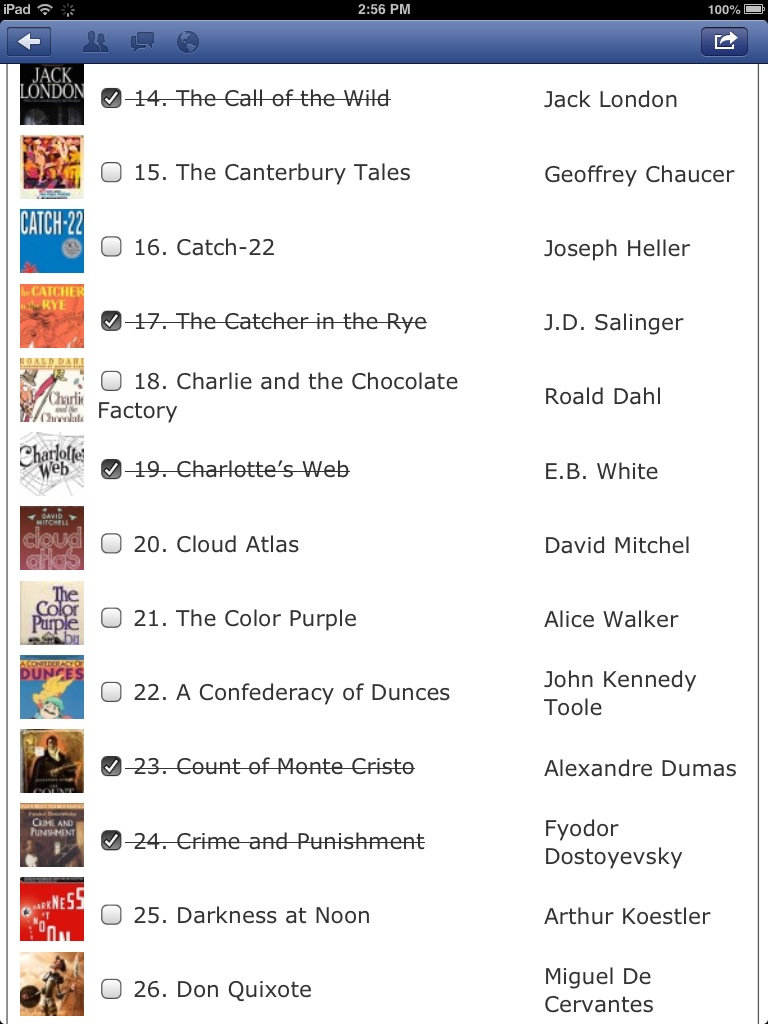The image appears to be a detailed screenshot taken from an iPad. At the top left of the screen, it reads "iPad" with a Wi-Fi signal and a loading icon next to it, indicating some activity. The time in the top center shows 2:56 p.m., and the top right corner indicates that the battery is fully charged at 100%.

The main content of the screenshot is a list of books, numbered from 14 to 26. Each book entry features, from left to right, a small image of the book cover, a check box, the book number, the book title, and the author’s name. Several books have been checked off, with the titles crossed out to signify they have been read. The following titles are crossed out:
- Number 14: "The Call of the Wild" by Jack London
- Number 17: "The Catcher in the Rye" by J.D. Salinger
- Number 19: "Charlotte's Web" by E.B. White
- Number 23: "The Count of Monte Cristo" by Alexandre Dumas
- Number 24: "Crime and Punishment" by Fyodor Dostoevsky

The unchecked and not crossed out books, along with their respective authors, are:
- Number 15: "The Canterbury Tales" by Geoffrey Chaucer
- Number 16: "Catch-22" by Joseph Heller
- Number 18: "Charlie and the Chocolate Factory" by Roald Dahl
- Number 20: "Cloud Atlas" by David Mitchell
- Number 21: "The Color Purple" by Alice Walker
- Number 22: "A Confederacy of Dunces" by John Kennedy Toole
- Number 25: "Darkness at Noon" by Arthur Koestler
- Number 26: "Don Quixote" by Miguel de Cervantes

The layout is clear and organized, with the text in black and some alternating colors like yellow, orange, blue, red, brown, and white in the book cover images, giving it a colorful appearance.